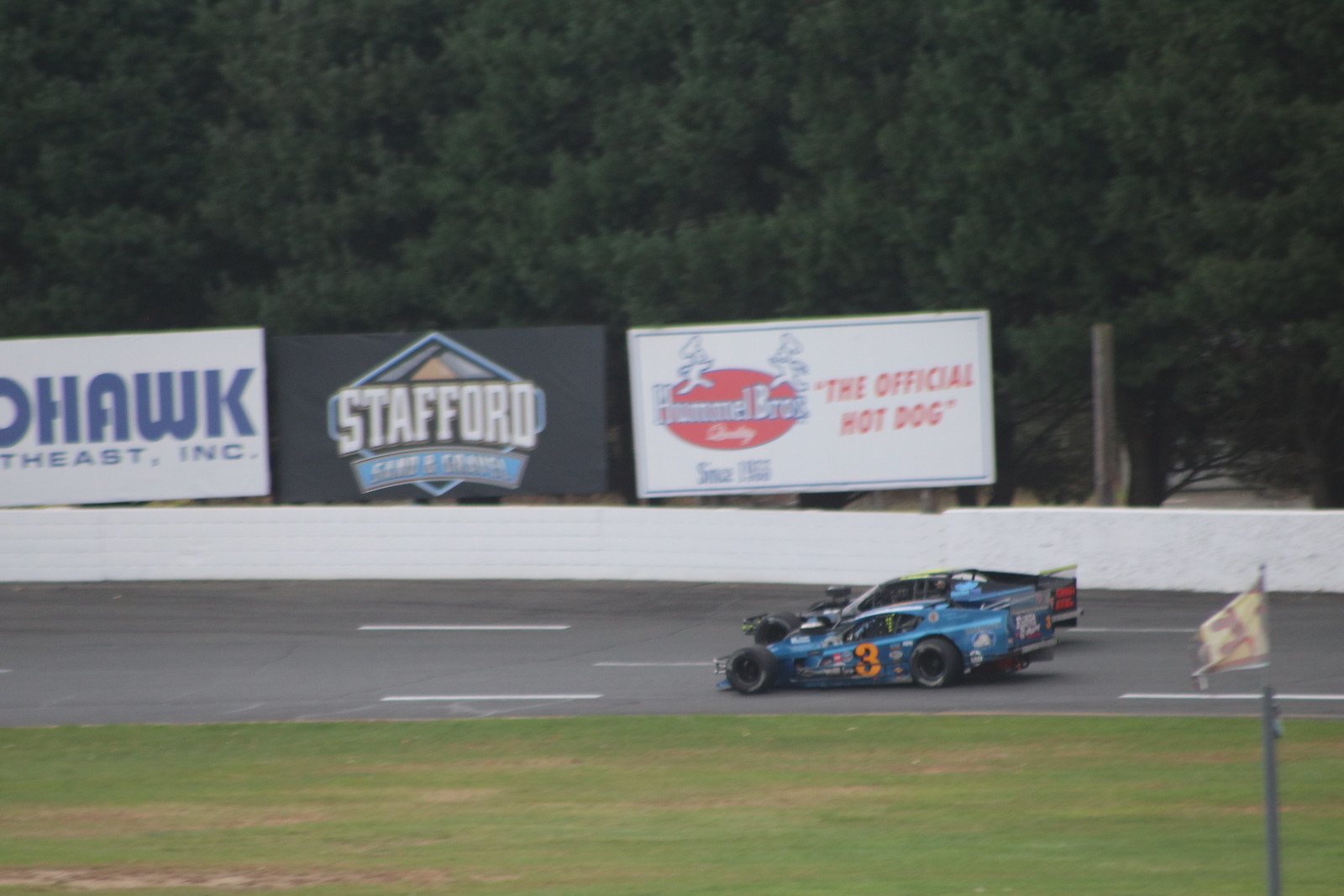In this action photograph, we see two NASCAR race cars speeding side by side on the outside stretch of a track. The car in the foreground is blue with an orange number three, while the car trailing it appears to be black with yellow accents. The cars are flanked on the left by the green grass of the infield and on the right by a white barricade wall adorned with advertisements. Prominent among these ads are banners for Hawk Southeast Incorporated, Stafford, and Hummel Bros, the official hot dog. In the background, tall trees line the edge of the track. A flag, blowing in the wind, indicates that it is a windy day. Despite some blurriness, the photograph captures the high-speed nature of the race, with the moving flag emphasizing the dynamic setting.